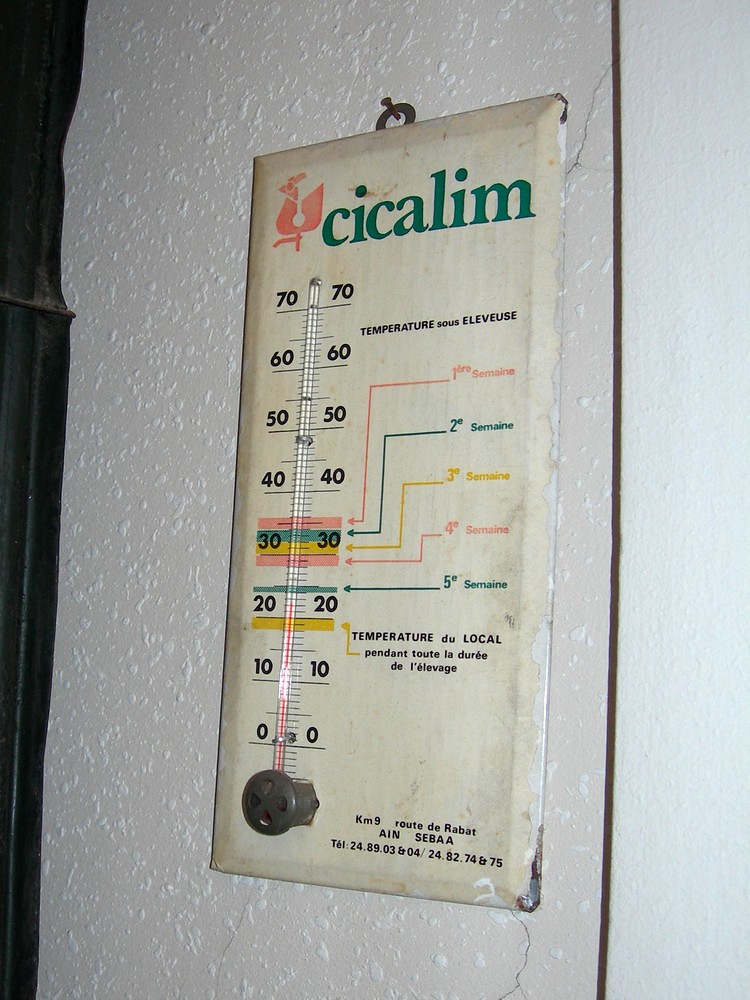This vibrant color photograph captures a metal thermometer mounted on a wall, secured by a nail. The thermometer features inscriptions in French and is adorned with a charming illustration of a rooster at its top, accompanied by the word "cyclam." The temperature scale, marked in increments of 10 degrees from 0 to 70, runs vertically along the device. To the right of these markings are colorful arrows indicating various temperature-related annotations.

At the top-right, just below the 70-degree mark, the text "temperature sous-elevus" is inscribed, followed by the term "1ere semaine" (1st week) in pink. Progressing downward, "2e semaine" (2nd week) is highlighted in green, "3e semaine" (3rd week) in yellow, "4e semaine" (4th week) in pink, and "5e semaine" (5th week) again in green, each pointing to their respective temperatures. At the bottom, the text "temperature du local pendant la durée de l'élevage" provides context, indicating the local temperature during the breeding period.